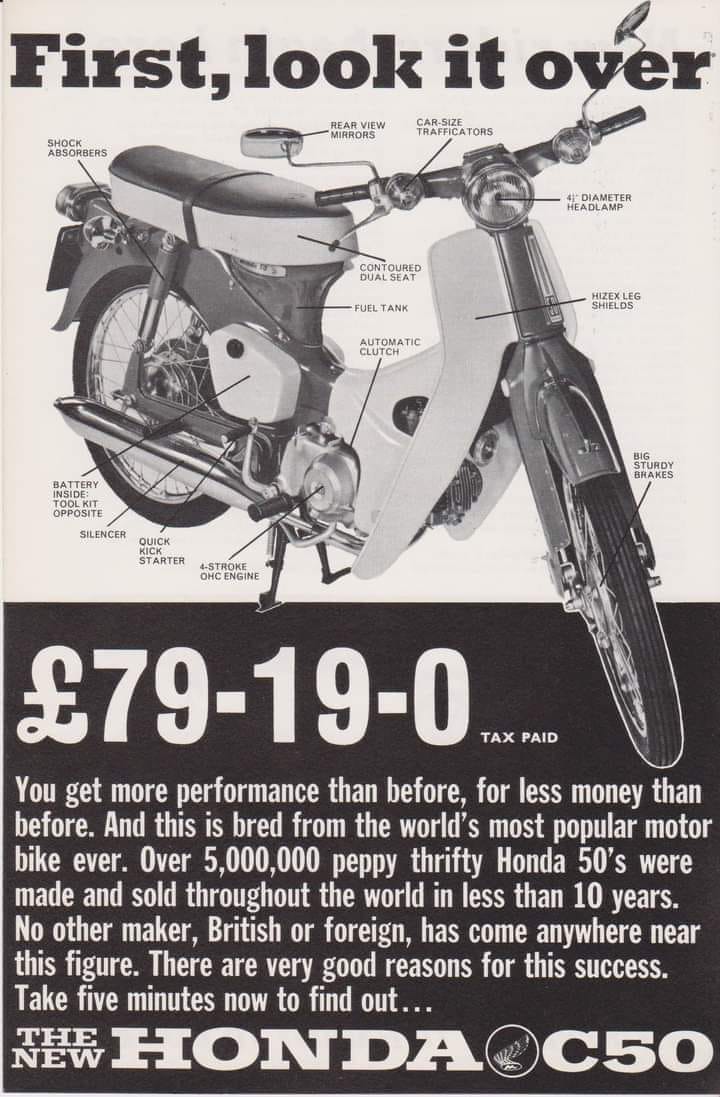This vertical black-and-white advertisement for the new Honda C50 motorbike, set against a primarily whitish gray background with darker smudges near the upper right edges, features a detailed layout reminiscent of a manual or paper. The top portion of the ad contains bold black letters proclaiming "First, look it over." Immediately below this text is a meticulously labeled image of the Honda C50, showcasing its long, flat seat with a black top. Various parts of the motorbike, including the shock absorbers, battery, tool kit, silencer, quick kick starter, 4-stroke OHC engine, big sturdy brakes, his X leg shields, contoured dual seat, fuel tank, automatic clutch, 4-inch diameter headlamp, car-size trafficators, and rear view mirrors, are distinguished with arrows and labels. Transitioning to the bottom section, the background shifts to solid black with white print detailing the bike's price as £79-19-0, with "tax paid" noted in smaller letters to the right. The left-aligned paragraph extols the virtues of the Honda C50, emphasizing its superior performance and affordability, attributing its design to the wildly successful Honda 50, which sold over five million units globally in less than a decade. The text underscores the unmatched success of the Honda 50 compared to other motorbike makers. The advertisement culminates with the bold, stacked text "The new" followed by "Honda C50" in large white letters.